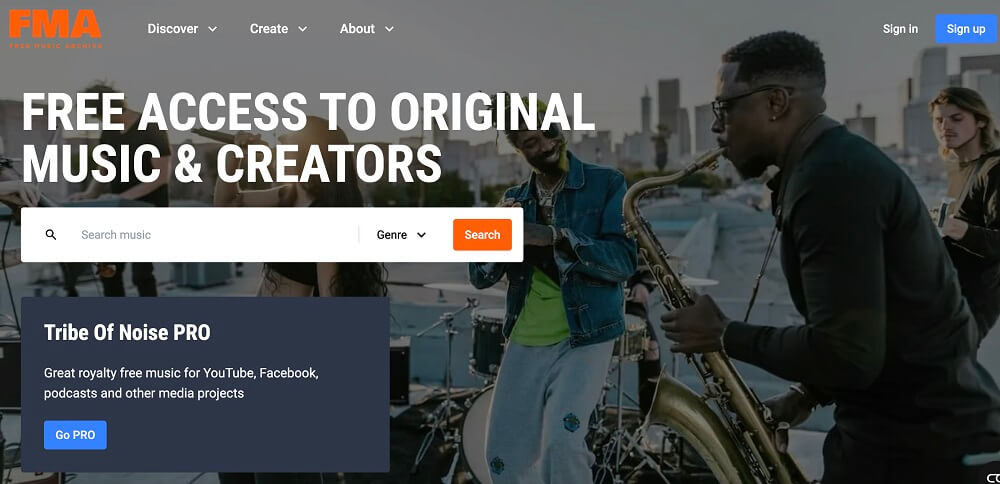Screenshot of the FMA website, a company specializing in providing original music and content creators for YouTube, Facebook, and other media platforms. The website's logo is located in the top left corner with the initials "FMA," though the full name is not clearly legible. Adjacent to the logo, there are navigation headings including "Discover," "Create," and "About." 

In the top right corner, there's a user access panel featuring "Sign In" and "Sign Up" options, the latter highlighted in blue with white text. Dominating the left side of the screenshot is a bold, prominent message: "Free access to original music and creators." Beneath this text is a search bar labeled "Search music," accompanied by a magnifying glass icon, a genre dropdown menu, and an orange search button.

At the bottom left, there's a text box titled "Tribe of Noise PRO," which describes itself as offering "great royalty-free music for YouTube, Facebook, podcast, and other media projects." It includes an option to "Go Pro" for access to higher-quality or more comprehensive music options, likely for a fee.

The background image showcases a group of young men engaged in music creation, with one prominently playing a saxophone at the forefront. The setting appears to be outdoors on a hazy, gray day, with a faint city skyline in the background.